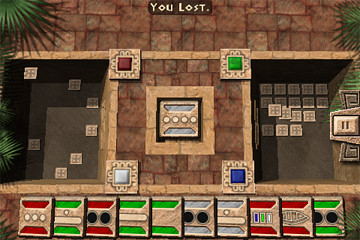This detailed colour illustration seems to depict a scene from an unfamiliar game. At the top of the image, there is a brown paved area interspersed with patches of green foliage in the right and left corners, creating a rugged, natural border. 

Centrally positioned at the top is a black sign with white text that reads "You Light." Below this sign, there lies a lighter brick square, subdivided into smaller quadrants. Each corner of this central square features a differently coloured section: blue, dark red, green, and dark blue, adding a vibrant contrast to the scene.

Flanking this lighter brick square are two darker greyish squares on either side, each scattered with what appear to be tiny playing cards casually placed within them. These darker sections create a sense of symmetry and balance in the layout.

At the bottom of the illustration, there is an array that resembles a line of slot machines, adorned in vibrant shades of red, green, and blue. These machines add an element of intrigue and playfulness to the scene, although their exact function within the context of the game remains ambiguous.